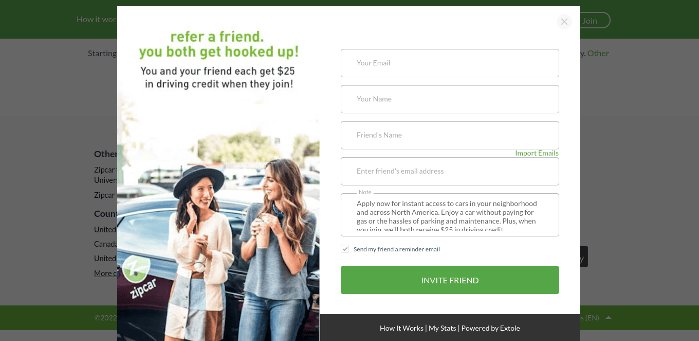The image displays a website with both the top and bottom portions of the background showing green banners. However, this background is muted due to an overlaying pop-up. The pop-up features a white background and prominently showcases a referral offer.

At the top of the pop-up, there is green text in lowercase letters that reads, "refer a friend. you both get hooked up!" Below this, a line of black text states, "You and your friend each get $25 in driving credit when they join."

Beneath the text, there's an image featuring a car and two women, standing side by side, leaning on the car. The car has a graphic of a green circle with a "Z" inside it and the word "Zipcar" written underneath.

On the right side of the pop-up, there are fields for user input labeled "your email," "your name," "friend's name," followed by a green text option saying "import emails". Below these fields, there is a section to enter the friend's email address. Additional descriptive text is partially visible but cut off, suggesting benefits of the service like instant access to cars and perks such as not having to pay for gas or deal with maintenance. 

A checkbox that accompanies the partially visible text reads, "send my friend's reminder email," and it is checked.

At the bottom of the pop-up, there is a blue (or green, based on conflicting description) banner with white text that says "invite friend". The muted black banner at the bottom of the overall image reads "how it works," "my stats," followed by "powered by XTOL."